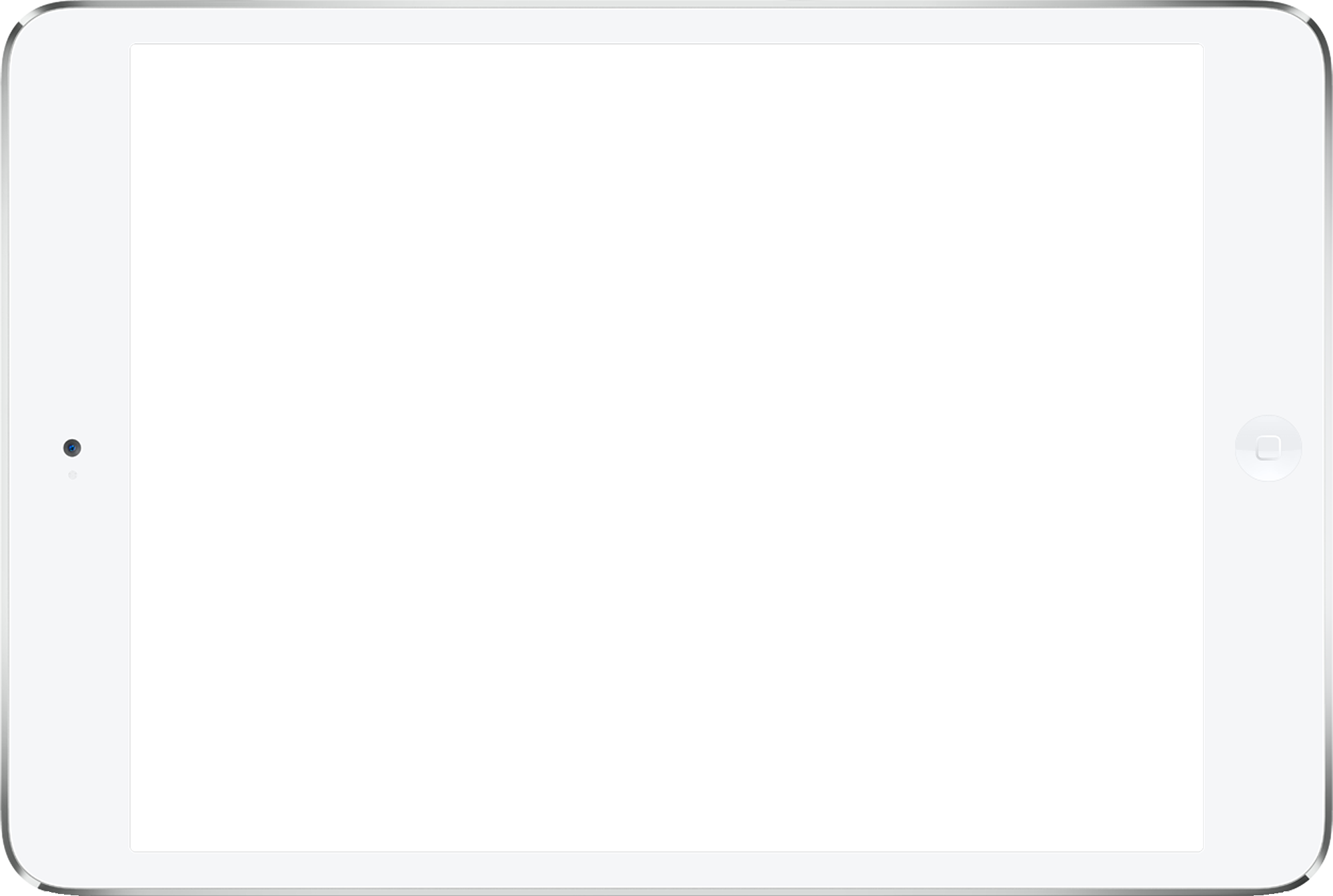A high-resolution image showcases a sleek, white tablet with a large, blank white screen, creating the illusion of the screen seamlessly blending into the similarly white background. The device is elegantly framed with a thin silver lining. Notably, a small, circular feature on the left middle edge suggests the presence of a camera or speaker, while the right side hosts a distinctive white button embedded with a square, typically used for home screen navigation or other functionalities. The overall clean and minimalist design, accentuated by subtle lighting on each corner, lends the photograph an almost illustration-like quality. The pristine presentation and flawless detail imply that this image likely serves promotional or marketing purposes, emphasizing the tablet's refined design.